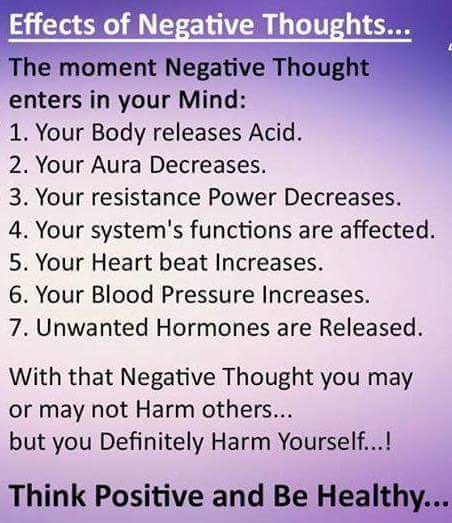The image features a rectangular poster with a gradient purple background that transitions from dark purple at the top to white in the middle and light purple at the bottom. At the top, the headline "Effects of Negative Thoughts" is written in bold white letters and underlined. Below this, in black text, it states: "The moment a negative thought enters your mind;" followed by a numbered list of consequences: 1. Your body releases acid. 2. Your aura decreases. 3. Your resistance power decreases. 4. Your system's functions are affected. 5. Your heartbeat increases. 6. Your blood pressure increases. 7. Unwanted hormones are released. A paragraph underneath reads, "With that negative thought, you may or may not harm others, but you definitely harm yourself." At the bottom of the poster, a bold black statement urges, "Think positive and be healthy."